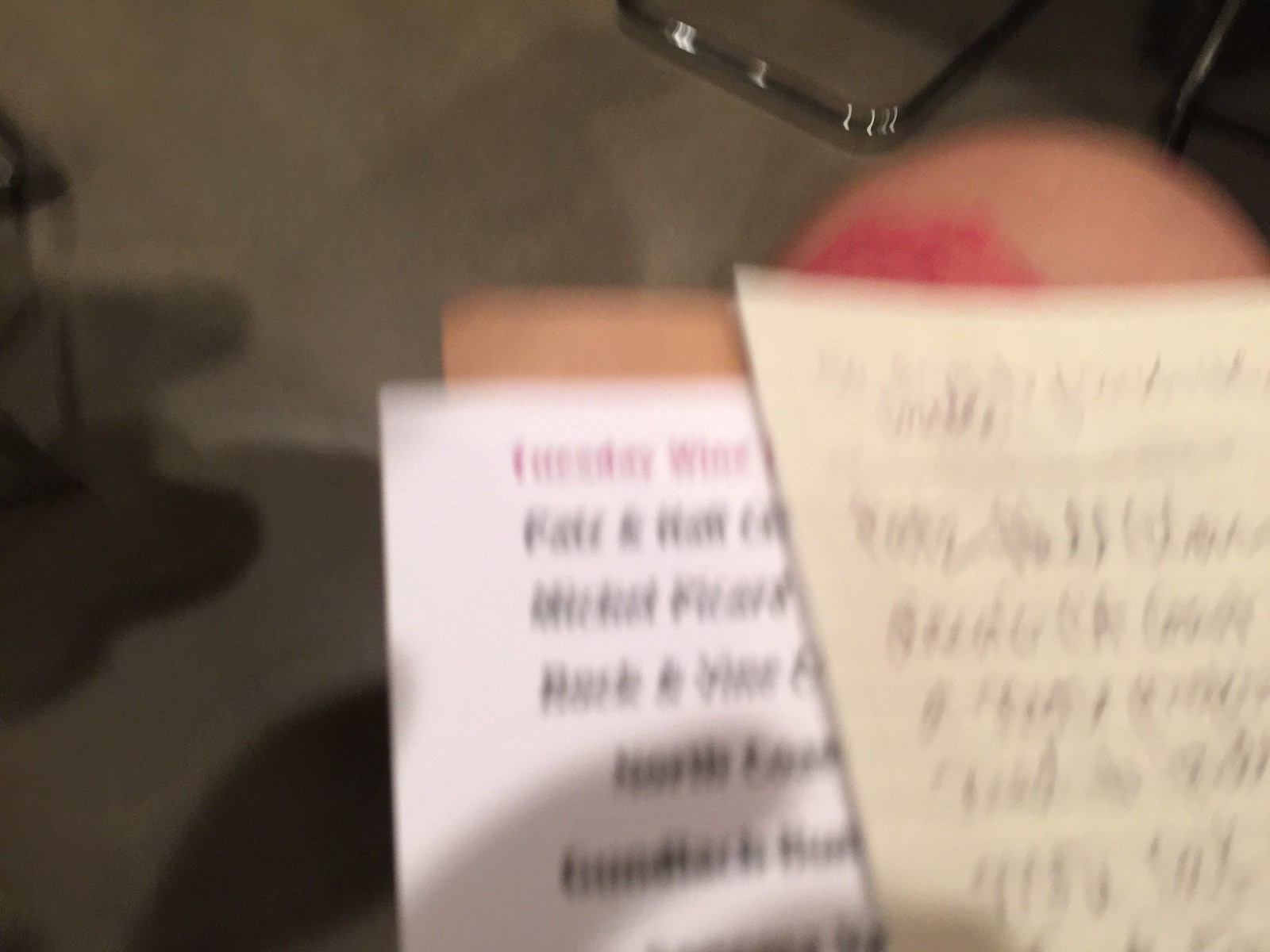This is an extremely blurry photograph set in a room, possibly inside a school classroom. The image appears to be taken from a perspective looking down at the edge of a desk or perhaps a person's lap. Off to the left of the image, there is some sort of black object that resembles a shelf, and the wall in the background is a gray color. In the top center, there is a metal bar or silver handle visible. In the foreground, there are two slightly overlapping pieces of paper. The piece on the left is off-white with black print and a red title, which appears to say "Tuesday Wine," though the text is indistinguishable due to the blur. The piece of paper on the right is white with handwritten words that are also too blurry to read. Additionally, the image shows the tip of a knee in the top right-hand side and possibly the floor and bottom of another desk.